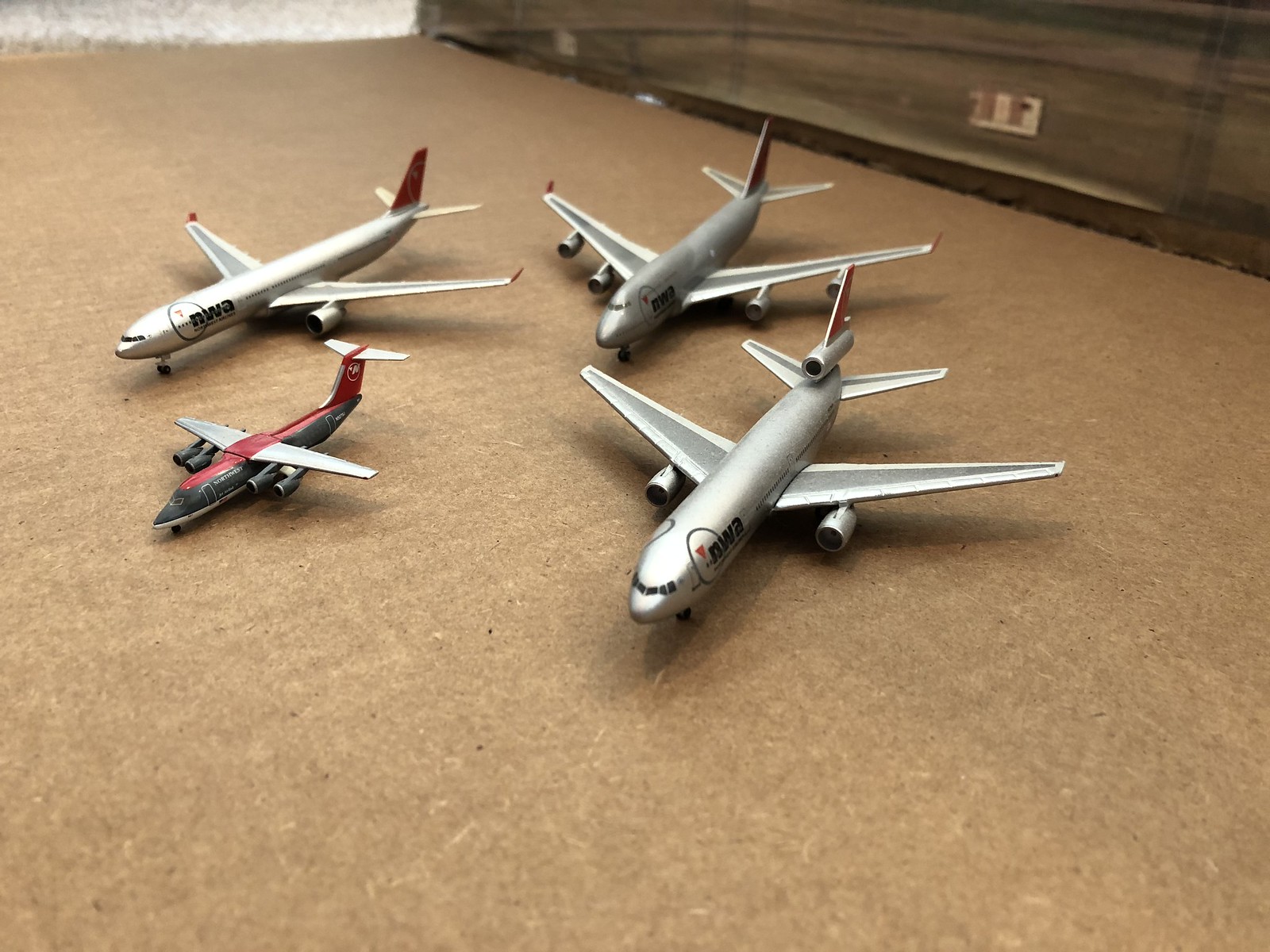This photograph showcases a collection of four small metal model airplanes, meticulously arranged on a light brown surface that resembles cardboard but might actually be a textured floor, possibly concrete. The upper left-hand corner reveals a portion of a dingy white wall with gray speckles, adding to the room's ambiance. To the right, a brown chest or dresser is partially visible, contributing to the background elements. The model airplanes predominantly feature a silver color with long wings and engines on either side. Three of the planes are similar in design, each bearing the NWA logo near the cockpit, indicative of passenger jets. The fourth plane stands out with its distinct black and red color scheme, being significantly smaller than the others. Notable shadows beneath the planes hint at a well-lit environment.